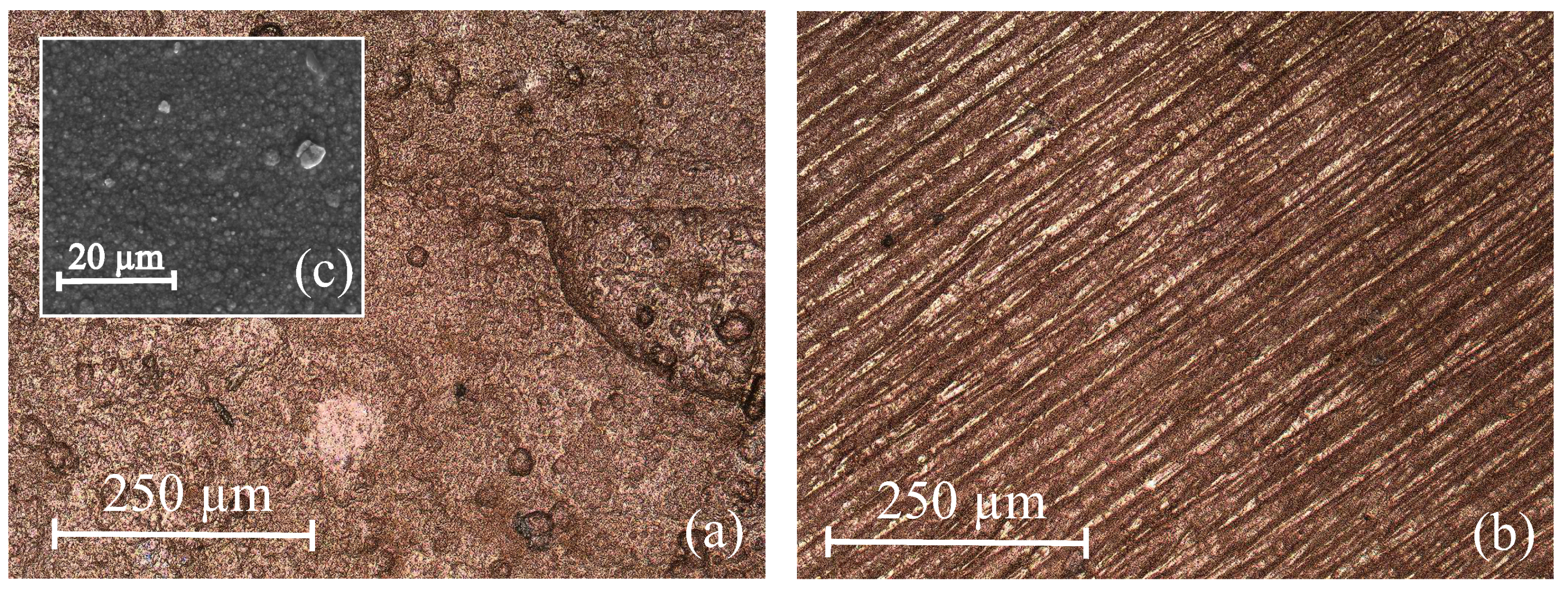This composite image consists of three microscopic views with a brown background, showcasing varying levels of detail and magnification. 

**Image A** (on the left) displays a highly irregular pattern comprising random circles and blobs in different shades of brown, with no apparent uniformity. The scale for this image is 250 micrometers, indicated in the bottom left corner. 

**Image B** (on the right) contrasts significantly with Image A, featuring a structured series of long, diagonal lines that stretch from the bottom left to the top right corner. These lines vary in shades of brown and are measured on the same 250 micrometer scale.

Inset within Image A is **Image C**, which is zoomed in further and depicts gray pebbles of varying sizes, reminiscent of dirt particles. This close-up view includes a scale of 20 micrometers.